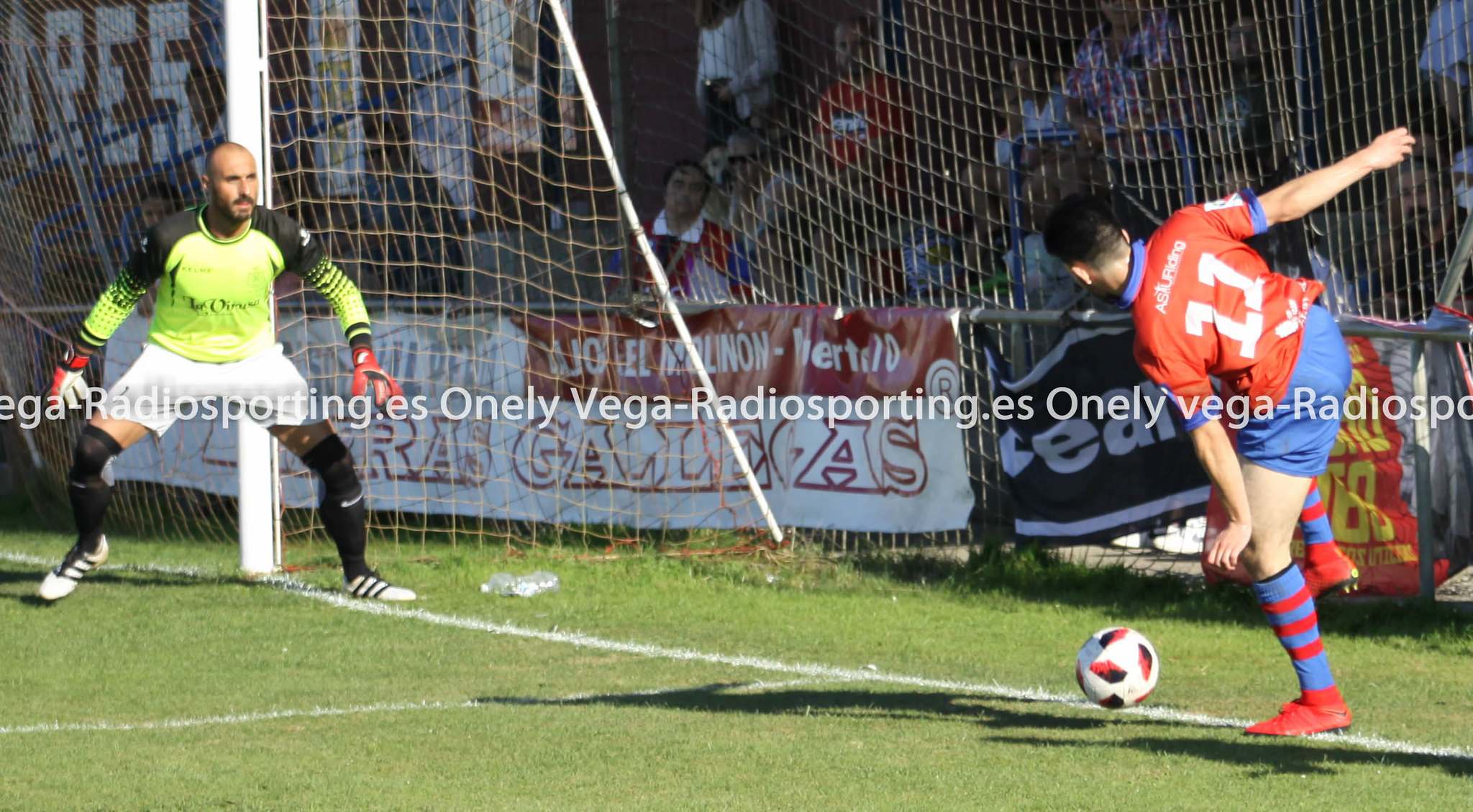The image depicts an intense soccer match scene, featuring two key players near the goal area. To the left stands the goalkeeper, dressed in a neon green and black shirt, white shorts, and high black socks, complemented by white and black cleats. His outfit is completed with thick red and white gloves as he stands alertly in front of the goal, facing the action to his right. The goalkeeper is bald, adding a distinctive look to his anticipatory stance.

On the right side of the image is another player, identified by his red jersey marked with the number 11 in white. He sports blue shorts and blue socks with red stripes, paired with red shoes. This player is caught mid-action, his right foot raised, poised to kick the ball positioned precariously on the end line, just about to go out of bounds. His right arm is extended to the side for balance, while his left arm hangs downward. 

Fans can be faintly seen behind the net, adding to the charged atmosphere as they watch the unfolding play with bated breath. The goal and part of the stands with some netting are visible, framing the intense moment. A watermark on the image reads "EGA radiospotting.es onlyvega-radiospottings.es onlyvega radiospo."